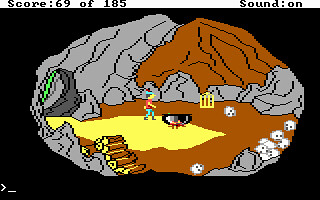The image depicts a scene from a vintage video game, reminiscent of those from platforms like Atari or Apple IIe. The aspect ratio of the image is approximately 1.5 times wider than it is tall, and the frame is entirely bordered in black. At the very top of the screen, there is a score display reading "Score: 69 of 185" on the left, and "Sound: On" in the upper right corner. The scene itself appears to be set inside a cave, characterized by a mix of gray and brown rock formations. 

In the center of the image, a male character is visible, dressed in a blue hat, red shirt, and blue pants. He stands near a campfire, over which a black pot or cauldron is hanging. Piles of wood are placed towards the bottom of the cave. On the left side, there’s what appears to be a cave entrance, while the back wall on the right features a treasure chest. Additionally, the far right wall is adorned with skull-like shapes.

Touches of color punctuate the rocky landscape: there’s some yellow in the center and silver rocks on the left side, giving the impression of a campsite in a rugged terrain. The game scene overall has various yellow details, including an indeterminate set of yellow bars or lines toward the far end of the cave background, alongside some other indistinct white details with black dots.